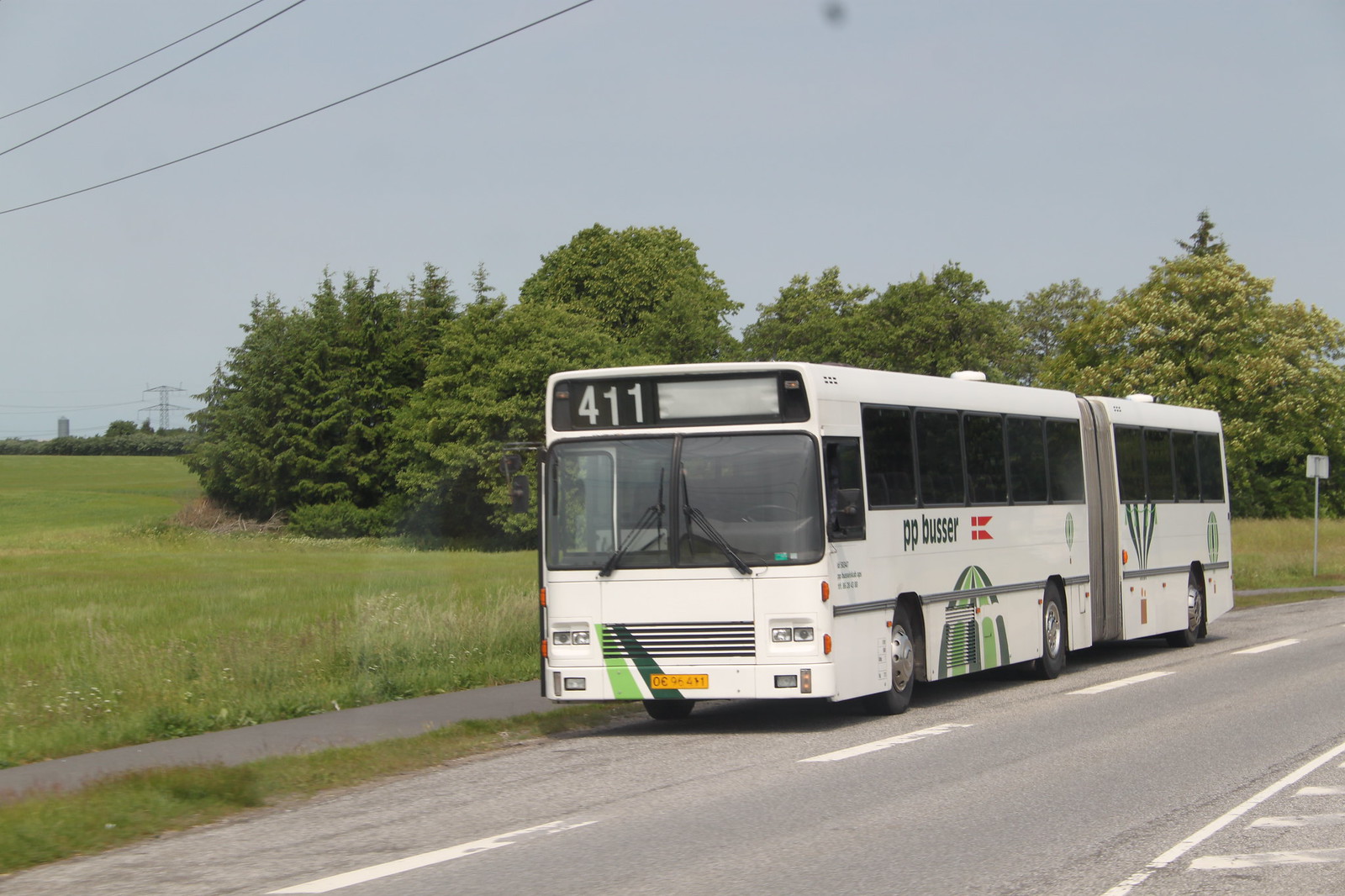A detailed photograph captures a large white city bus with the number 411, prominently defined by its dual-compartment structure—an accordion-like connector linking the main body and an extension section. The bus, emblazoned with the text "PP Busser" beside a red and white flag, features whimsical green and white hot air balloon designs scattered along its side. It is parked on the side of a broad, gray road, likely a highway, with no visible driver or passengers. The lush surroundings include fields of long green grass and tall, bushy evergreen trees stretching into the distance, encapsulating the countryside setting under a clear, blue-grey sky devoid of clouds. The photo is taken from a landscape orientation, offering a left-angled perspective of the bus on the middle right. In the far left, the field extends towards more trees, and a few power cables are visible in the top left corner, adding to the overall rural atmosphere.